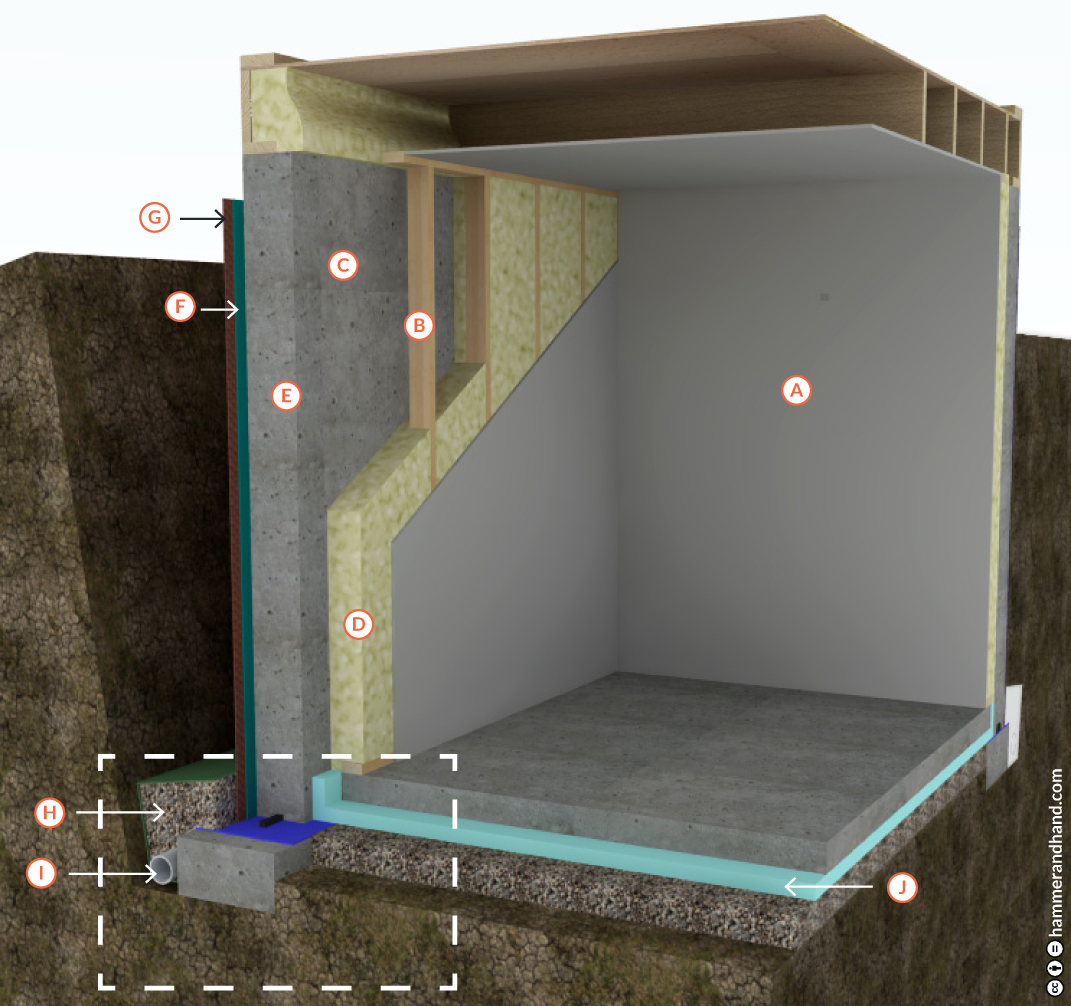The image is a highly detailed 3D graphic showcasing the foundation and internal structure of a building, possibly a home, a video game environment, or a shed. The main components of the building are meticulously labeled with red letters (A through J) inside white circles, which are scattered throughout the image. The foundation appears to involve various materials including wood, cement, and insulation, indicating different construction levels. The image also depicts the foundation extending into the ground, with the surrounding earth visible. Notably, there is a white dotted arrow box at the bottom of the graphic that highlights a pipe or tubing, which might represent a sewer system that is being integrated with the foundation. This tubing is confined to the lower left corner and is labeled with letters H and I, amidst a ground-like structure.